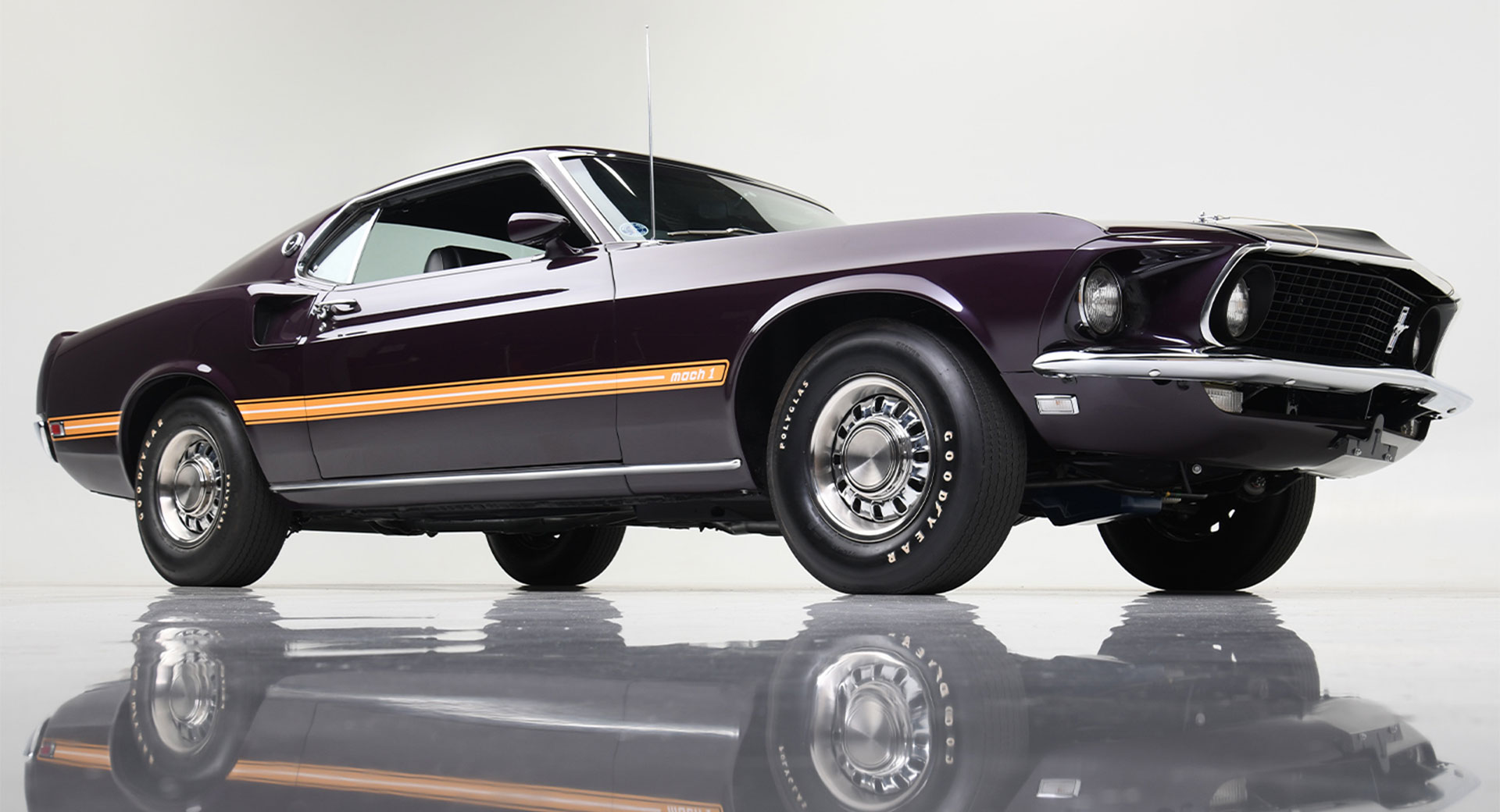This is a floor-level, portrait-oriented image of a pristine, vintage Mustang captured in profile. The classic car features a body painted in a striking combination of bright dark purple on the top and a lighter metallic purple below, separated by a vibrant yellow pinstripe running along the middle. Its chrome accents, including the window trim, door handles, bumper, antenna, and wheels, gleam brilliantly. The Goodyear-branded tires add a touch of authenticity to the meticulously maintained vehicle. The car rests on an exceptionally shiny white floor, mirroring its elegant form. The background is a soft whitish-gray, allowing the car's vivid colors and detailed craftsmanship to stand out.